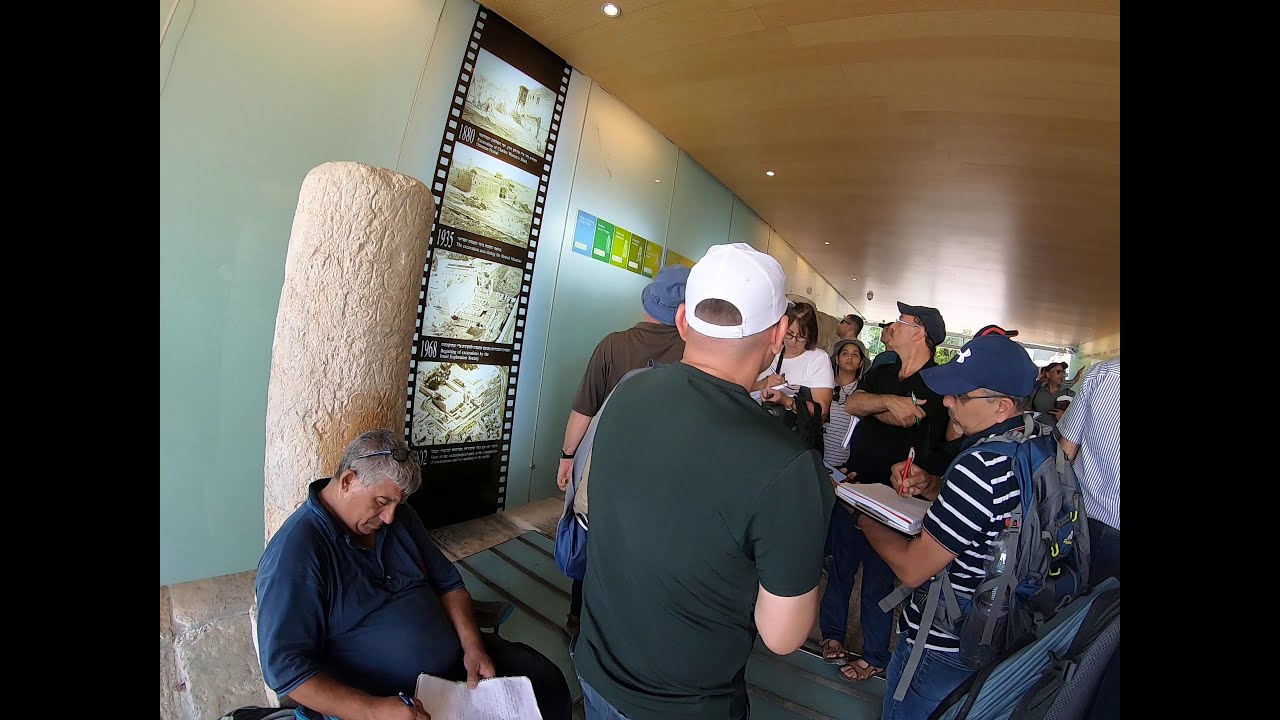In this photograph, you see a group of people, both men and women, gathered in a narrow room that almost resembles a hallway. The ceiling is smooth wooden paneling with inset lights. On the left side of the image, there is a pale blue wall running diagonally from top to bottom, adorned with a series of four slides that look like an old strip of film, each featuring an image with captions underneath, suggesting they explain something important. Next to the slides, there is a large white stone pillar. Most individuals are standing, engrossed in the slideshow, while a few are making notes. Particularly noticeable is a man on the bottom right who is wearing a blue and white striped shirt, a blue baseball cap, a blue backpack, and is jotting down notes in a notepad with a red pen. Another man is seated towards the front of the picture, dressed in a blue shirt, also focused on writing on a piece of paper. The whole scene conveys an intense focus on the information presented on the wall.